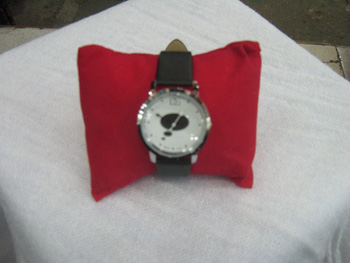This snapshot color photograph captures a small, red hand-sewn pillow at the center of the composition, resting on a diagonal-shaped table draped with a slightly wrinkled white cloth. The table’s edges are cut off, extending beyond the frame, with a backdrop featuring a tile floor and a dark brown wall. At the heart of this image, a wristwatch is wrapped around the pillow. The watch features a white clock face with a horizontal black oval in the center and is adorned with dark brown leather straps running north and south. Though the face of the watch is slightly out of focus, hints of the minute and hour hands are visible, along with faint numbers and glossy highlights reflecting light from above.